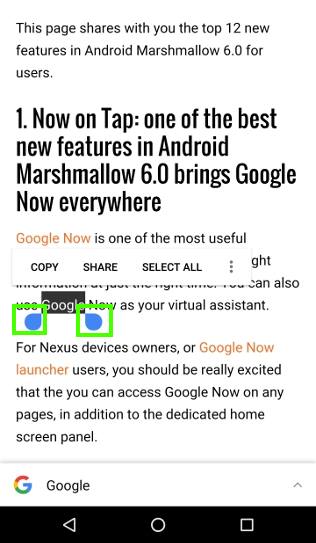A screenshot taken from an Android smartphone highlights a portion of a webpage discussing the top 12 features of Android Marshmallow 6.0. The distinct aspect ratio of the image, being notably taller than it is wide, as well as the presence of typical Android navigation icons—a back-facing triangle, a central circle, and a square on the right—confirm the device type.

Central to the screenshot is a text-heavy webpage. At the top, a header reads "This page shares with you the top 12 features in Android Marshmallow 6.0 for users." Below this, the main body features a prominent heading that reads, "One. Now on Tap, one of the best new features in Android Marshmallow 6.0 brings Google Now everywhere."

The user has highlighted the word "Google" within this section. The highlighting is accentuated by two blue adjustment markers, each framed by a green square, indicating that the text can be expanded or contracted to select more or less content. Just above the highlighted word are the options to "Copy," "Share," and "Select All," providing quick actions for the selected text.